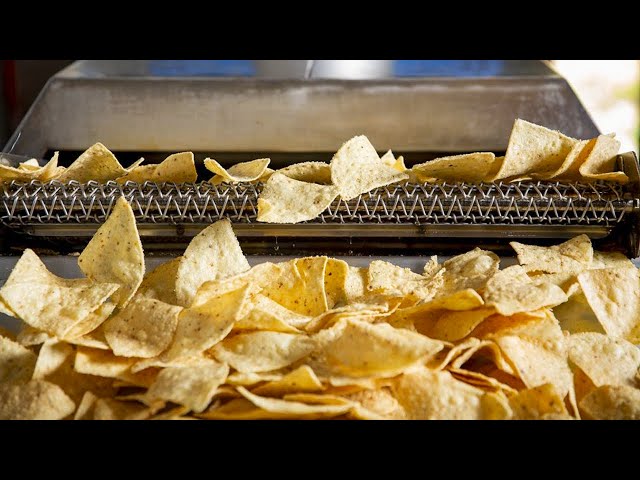The photograph depicts an industrial indoor setting with a very dark backdrop, where a metal machine is processing tortilla chips. The primary focus is on the silver machinery, which features an upper component resembling a cover or an elongated, oblong pan. The chips are being conveyed out from this silver-topped section on a chain-link style conveyor belt. Below this upper section is a lower tray or shelf where the chips are gathered. The tortilla chips appear to be white with black specks and are neatly aligned in a rectangular format as they fall from the conveyor, scattering in front of the machine. The overall scene is well-lit, highlighting both the chips and the machinery amidst the predominantly black background. No text or signatures are visible in the image, keeping the focus on the industrial nacho-making process.